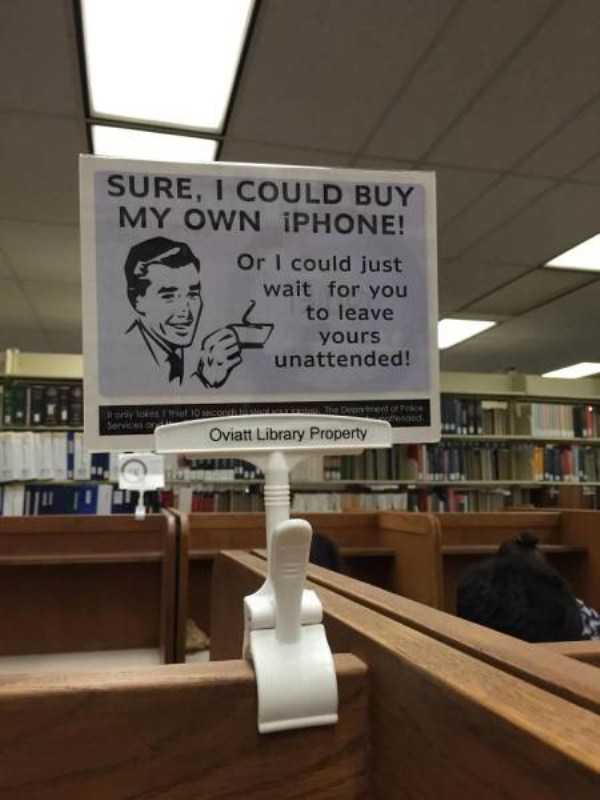The photograph, taken inside a library, showcases an arrangement of bookshelves filled with an eclectic mix of binders, tall books, and multicolored volumes lining the back wall. The ceiling, visible in the upper left part of the image, features white or gray tiled panels and fluorescent lights covered with plastic shields. In the foreground, a medium brown wooden cubicle desk is seen, to which a rectangular sign is clipped using a white plastic clip. The sign, framed by a white border and set against a gray background, bears the black text: "SURE, I COULD BUY MY OWN IPHONE, OR I COULD JUST WAIT FOR YOU TO LEAVE YOURS UNATTENDED!" At the lower left corner of the sign, there is an illustration of a smiling man in a suit jacket and tie, holding a cup of tea. Beneath the sign, on the clip's base, the text "Oviatt Library Property" is clearly displayed, indicating its ownership. The overall setting is that of an academic or public library, bustling with silent activity.